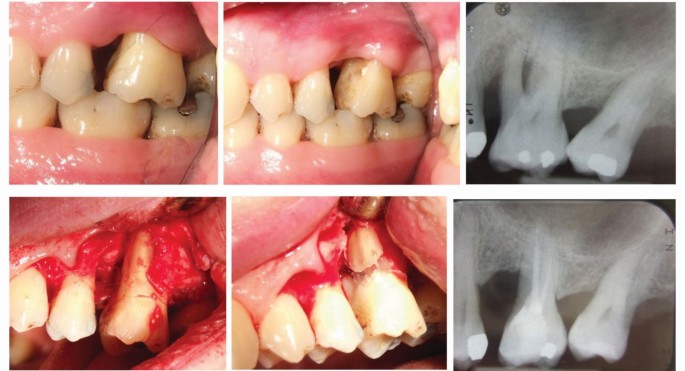This image is a detailed collage of six different photographs showcasing varying dental conditions and procedures. The images are arranged in two rows of three. Starting in the top left, the photograph depicts jagged, misaligned teeth with light pink exposed gums; a small implant or filling is visible on the far right tooth. The top middle image, slightly zoomed out compared to the first, shows off-white teeth with light to dark pink gums. The top right photo is a black-and-white x-ray of the front molars, revealing white spots and multiple fillings. 

In the bottom row, the leftmost image highlights highly inflamed, bloody gums surrounding the teeth, indicating a severe gum condition. The bottom middle photo also displays bloodied gums but from a different angle, showing dental surgical tools in action. The bottom right image is another black-and-white x-ray, presumably post-surgical, revealing reduced extra tooth material compared to the top right x-ray and showing multiple fillings. The x-rays provide a deeper insight into the dental issues, while the color images emphasize the visual and medical severity of the oral conditions.